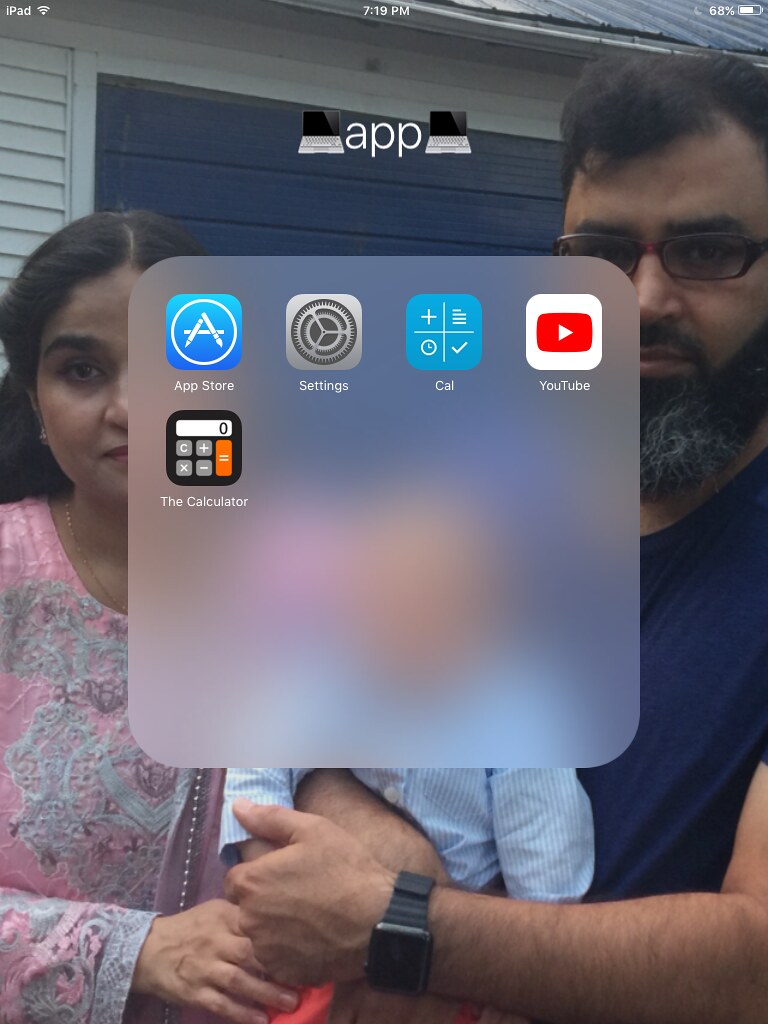A detailed view of a smartphone's home screen is captured in this image. At the top-left corner, "iPad" is displayed, while the center reads "7:19 PM," and the top-right shows the battery status at "68%" with an accompanying icon. The screen showcases several app icons, including the App Store, Settings, Calculator, and YouTube, in an organized layout. 

Beneath these app icons, a family photograph is partially obscured, revealing a man, woman, and their blurred child. The background of their photo features a blue garage door and a house, suggesting they might have recently moved in. Both adults are adopting serious expressions; the man, who seems to be holding the child, is wearing a short-sleeved shirt and a square smart watch, possibly a Fitbit. The woman, dressed in a pink embroidered dress, stands beside him. The photograph captures a moment in their lives marked by gravity and potentially new beginnings.